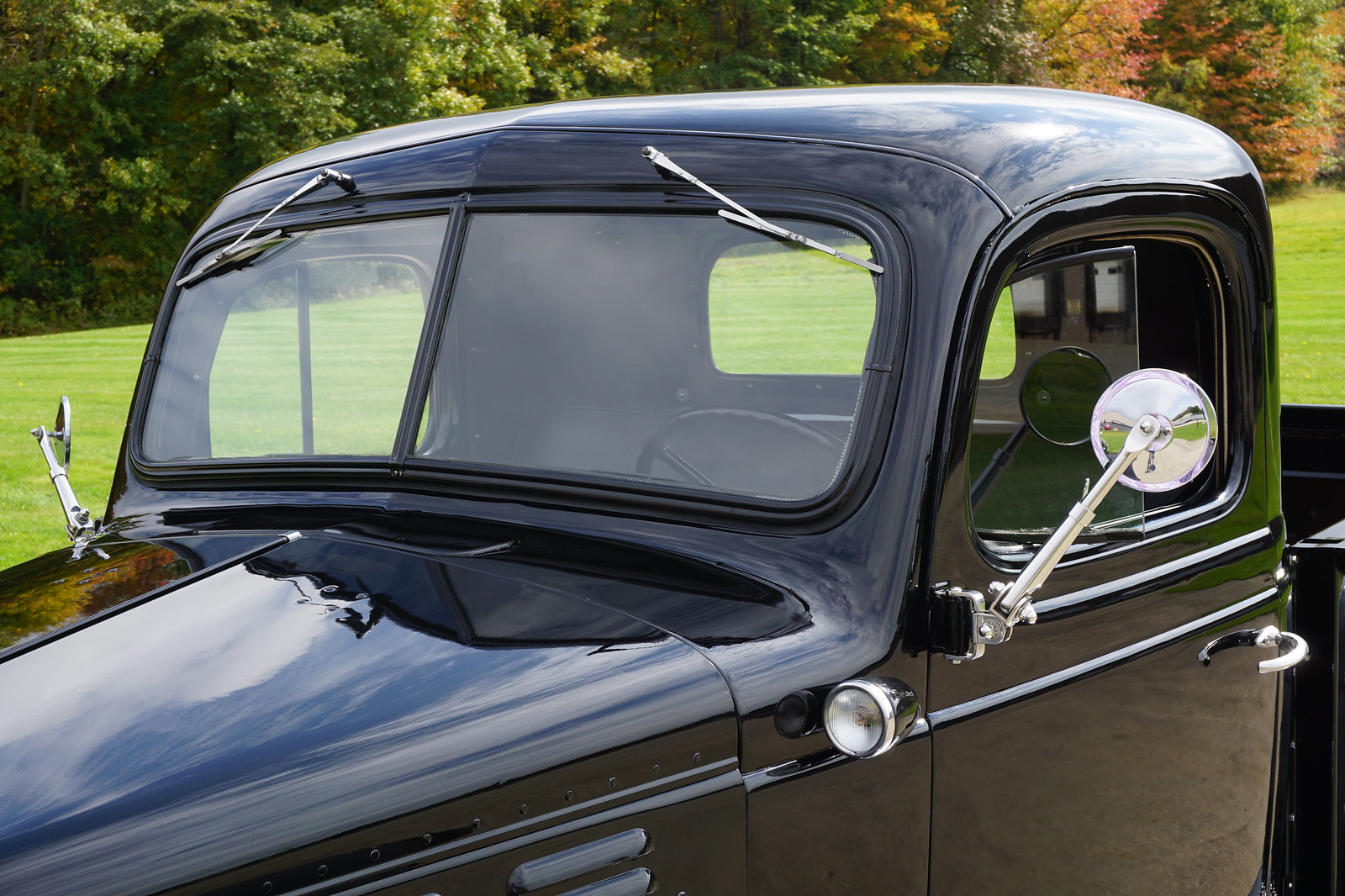This image captures a meticulously preserved, shiny black vintage truck, possibly from the early 1900s, estimated around the 1920s or 1930s. The truck, with its glossy waxed finish, displays an array of chrome accents, including two hanging windshield wipers, rearview mirrors on both sides, handles, and small lights on the sides. It boasts a cabin with square windows and a divided windshield. The truck's hood has a distinctive triangular shape, wider near the windshield and narrowing towards the front. Set against a backdrop of grassy expanse edged by autumnal trees, the image highlights not just the vehicle's well-maintained exterior but also reflections of the trees and sunlight shimmering on its surface. The scene suggests a tranquil fall setting, perfectly complementing the classic allure of this black Model T-like truck.